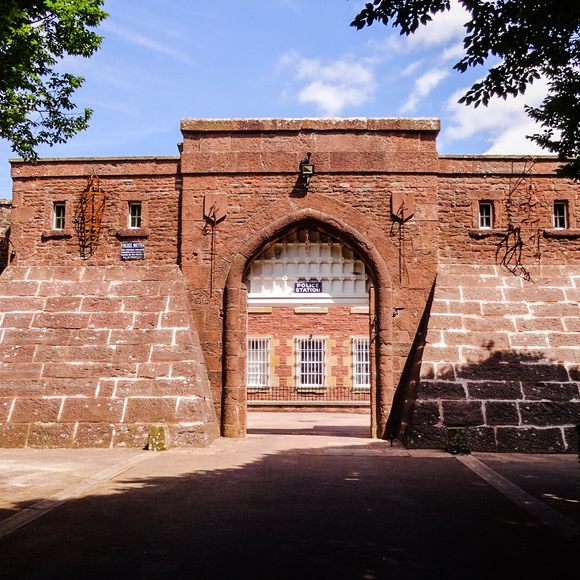The photo portrays a daytime scene of a brick police station characterized by large red and reddish-brown bricks making up its façade. Prominently at the front, an arched doorway sits at the top, positioned centrally under a large black sign with "POLICE STATION" emblazoned in white capital letters. Security measures are evident with a camera mounted on top of the building. The upper part of the building features two windows on either side, each with white bars that hint at the building's secure nature, possibly suggesting a jail or detention area.

The surroundings include a spacious walkway captured from the perspective of a sidewalk shaded by two trees, one on either side of the building. The clear afternoon sky with white clouds serves as a serene backdrop to the scene. The overall appearance of the structure presents a slightly aged and rustic feel, with some powdering and rusting visible on the brick walls. The image, devoid of any people, gives an impression of an empty or less active premise, contributing to a somewhat isolated atmosphere. The trees cast soft shadows onto the cement walkway, enhancing the peaceful yet stoic ambiance of the scene.